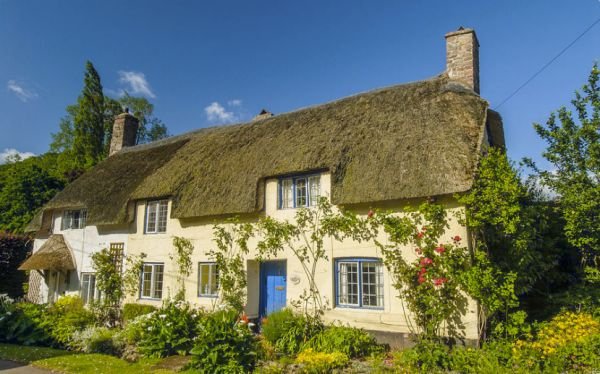Under a clear blue sky adorned with wispy clouds on the left, stands a picturesque, two-story, light tan house that exudes a charming, almost cottage-like appeal, though it is quite wide and spacious. The house features a distinctive green thatched roof, which appears mossy and even gives the impression of having grass growing on it. This unique roof is complemented by two chimneys, one on each end. The front of the house showcases a bright blue door centered amongst four bottom windows with paned glass. Above, three additional windows mark the second floor. The garden that surrounds the house is abundant with greenery, including very green bushes, ivy climbing parts of the walls, and a variety of wildflowers in hues of red, yellow, and white. Some bushes are blooming with red and small white flowers, and vines and other small trees add to the verdant scene. An awning extends over a side entrance, and a glimpse of nearby grass and a sidewalk can be seen on the left, enhancing the homely and inviting atmosphere.